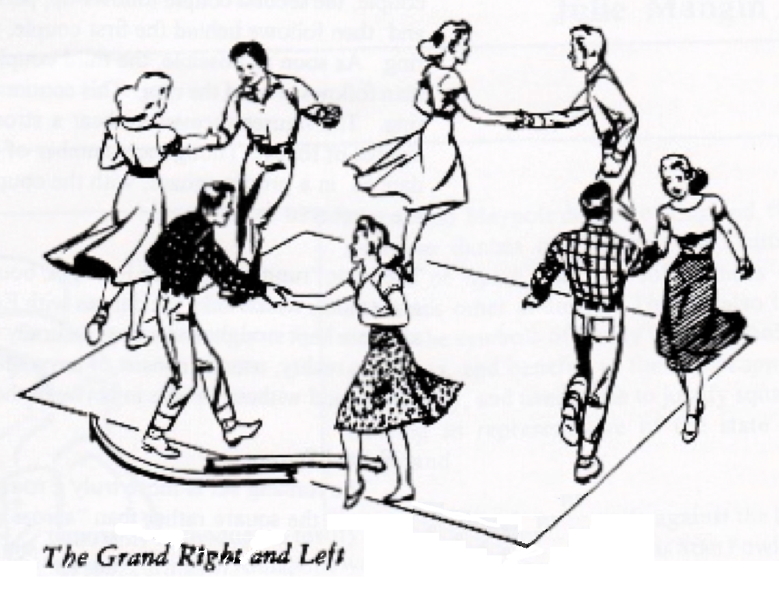This is a black and white pen and ink drawing depicting four couples engaged in a square dance, characterized by a caption reading "The Grand Right and Left" located on the lower left portion of the image. Rendered in a style reminiscent of the 1940s or 1950s, the dancers are captured mid-movement, each couple holding right hands. The women are dressed in long skirts and blouses, while the men don blue jeans, flannel or button-down shirts, and mostly cowboy boots. Notably, the dancers are arranged on a square dance floor diagram, with arrows at their feet indicating the direction of their movements, complementing the titled dance step. The simplicity of the drawing style balances detailed aspects such as the period-specific hairstyles and clothing. The facial features are minimally sketched, yet a few women are visibly smiling, adding a touch of joy to the scene.